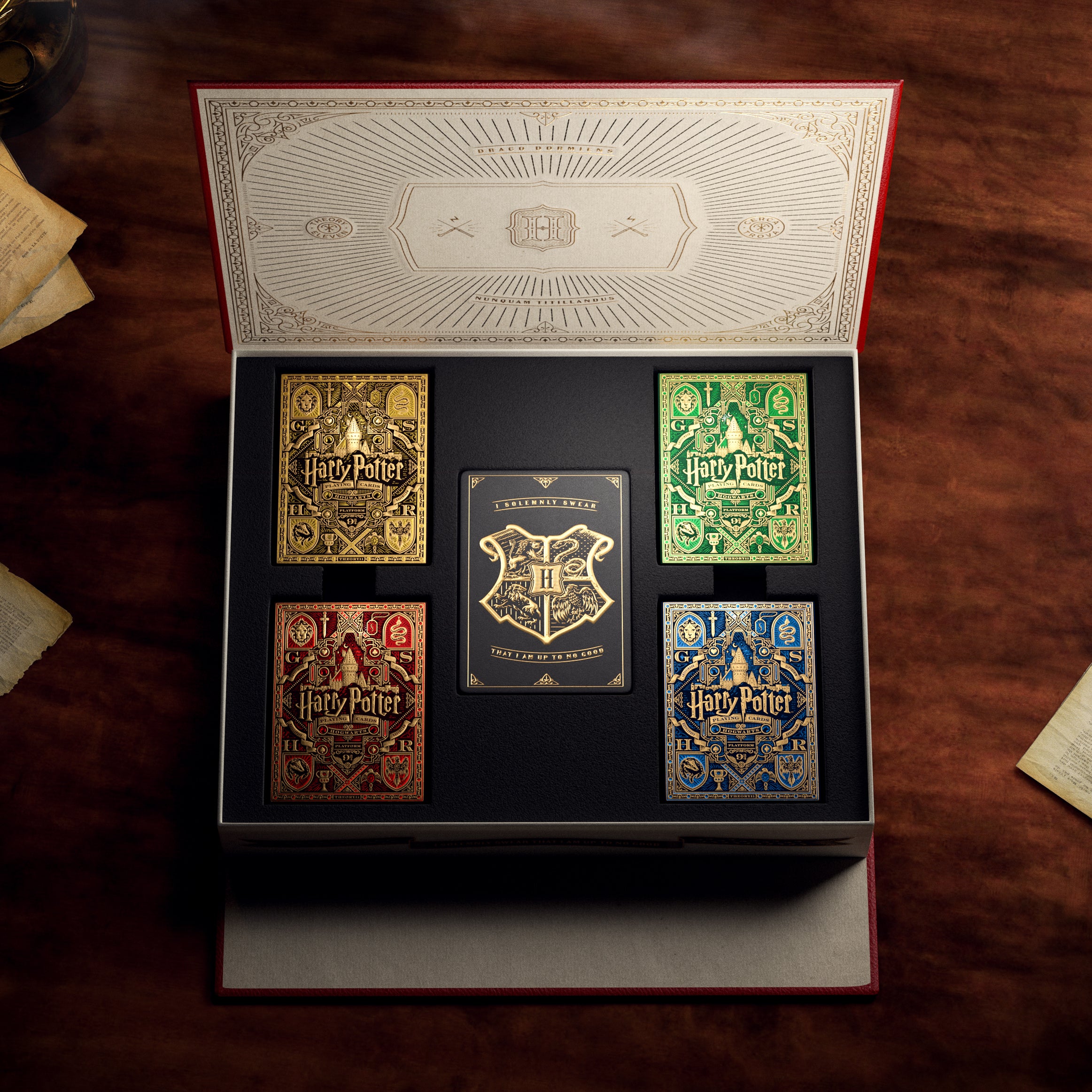The image is a square color photograph displaying an open box of collectible Harry Potter cards. The box has a white exterior with a red lid that features elaborate illustrations, including the phrase "I solemnly swear that I'm up to no good." Inside, the box has a black interior tray holding five distinct card-like objects. The cards are arranged in two rows with the central card standing vertically. This central card is black with a gold emblem featuring the Hogwarts Academy symbol, an 'H' encircled by intricate gold designs. Surrounding the central card are four other collectible cards, each with "Harry Potter" inscribed in the center and corner symbols representing the four Hogwarts houses. Clockwise, starting from the top left, the cards are colored yellow, green, blue, and red. The entire box is set on a dark wooden table.